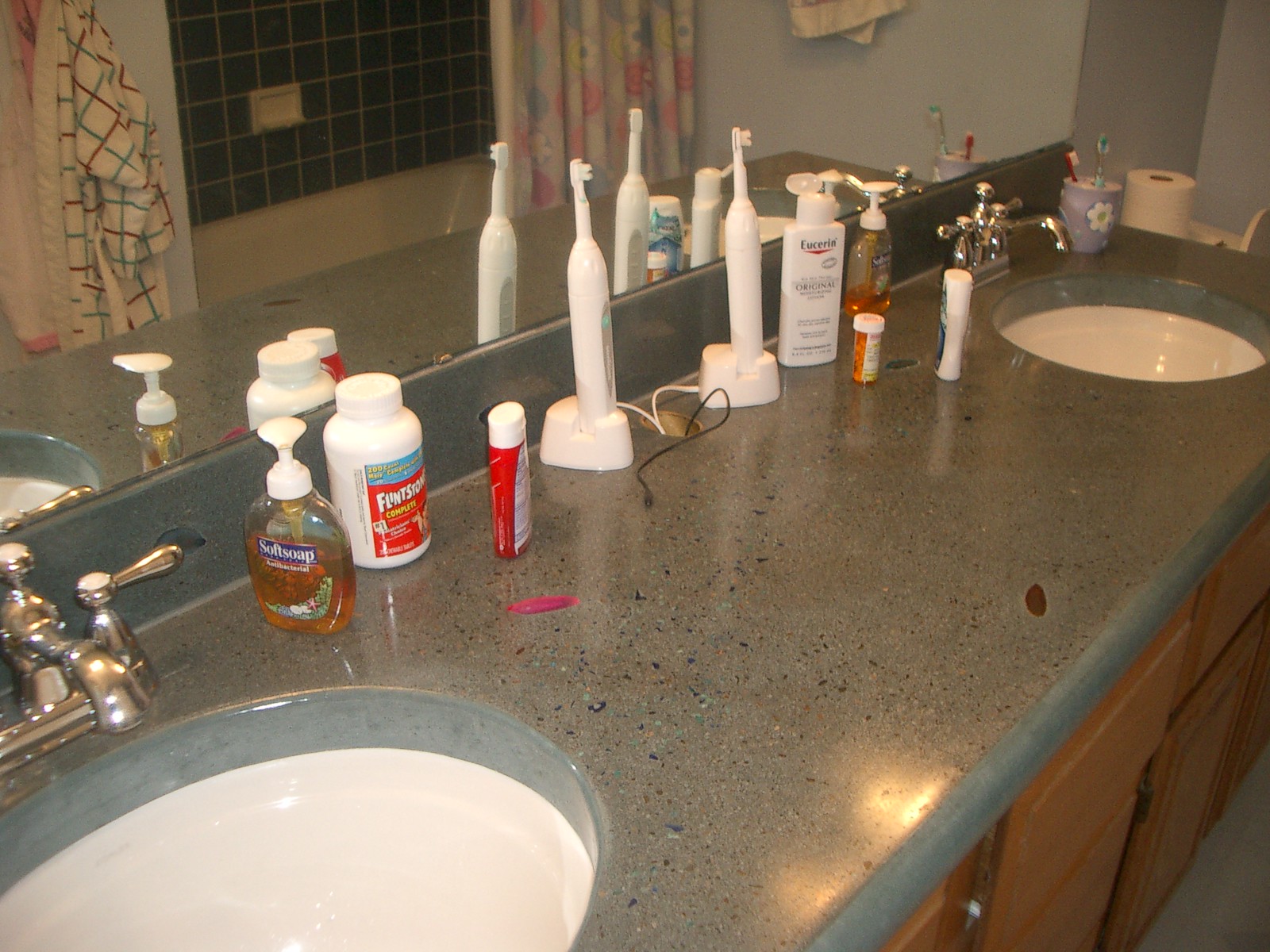This image showcases a spacious bathroom with dual sinks set into a lengthy, dark gray counter that features a speckled pattern of white, gray, and black. A large mirror is mounted above the counter, reflecting parts of the room. On the counter, various items such as toothbrushes, vitamins, hand soap, toothpaste, and prescription pills are neatly arranged, along with a toothbrush holder situated on the right end of the counter. 

Adjacent to the counter, a toilet is visible with a roll of toilet paper placed on top of the closed lid. The faucets and handles for both sinks are made of chrome, complementing the white basins. Below the counter, brown cabinets provide storage space, while the bathroom floor is a consistent gray color. 

In the mirror's reflection, several towels are seen hanging on towel holders; these include towels with white, red, and green stripes, as well as a pink and white towel. The shower area, painted green, features a white tub and is adorned with a colorful shower curtain.